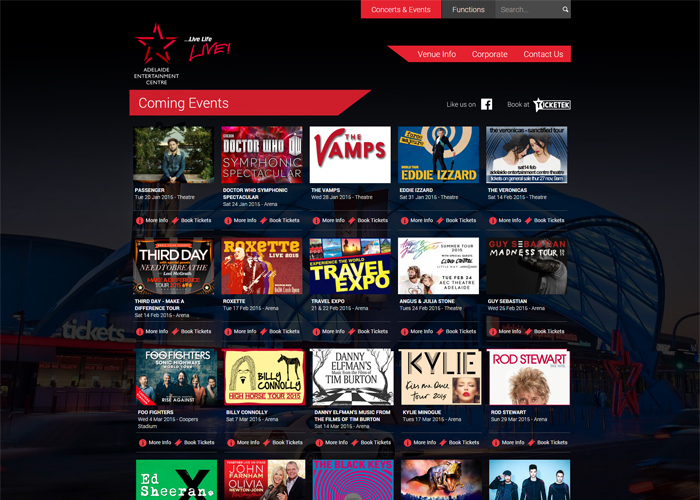This is an image of a website, presumably for a live entertainment center, albeit with poor resolution. The upper left corner of the website displays the name "Live Live Live" twice in white text and once in red text, alongside a red star. The text "ADLAJDE Entertainment Center" follows this emblem.

On the right side of the webpage, there are navigation options that include "Concerts and Events," "Functions," "Search a Venue," "Information," "Corporate," and "Contact Us." There are also social media prompts such as "Like us on Facebook" and booking information, encouraging users to "Book at Ticketex."

The section titled "Upcoming Events" lists an array of scheduled activities. This section comprises three complete rows and a partially visible fourth row, each containing five items. The first event listed in the top left corner is "Passenger," scheduled for Tuesday, June 26, 2015, in the theater. Adjacent to this, the next event is "Dr. Who Symphonic Spectacular," taking place on Saturday, January 24, 2015.